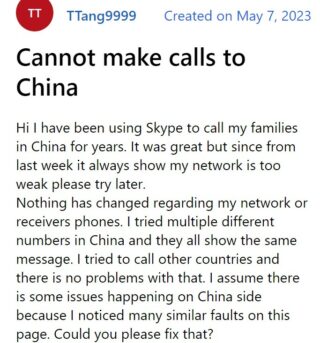Screenshot Description:

The image displays a portion of a web page, presumably a forum post. In the top left corner, a red circular icon contains bold white capital letters "TT." Adjacent to this icon, in hyperlink blue text, the username "TTANG" is visible, followed by the number "9999."

Below the username, additional blue text indicates the post's creation date: "May 7, 2023." The main content begins with a bold black heading: "Cannot make calls to China."

The body of the post, written in regular black text, reads:

"Hi, I have been using Skype to call my family in China for years. It was great, but since last week it always shows 'Your network is too weak, please try later.' Nothing has changed regarding my network or the receivers' phones. I tried multiple different numbers in China and they all show the same message. I tried to call other countries and there are no problems with that. I assume there are some issues happening on China's side because I noticed many similar faults on this page. Could you please fix that?!"

The image is cut off on all sides—top, bottom, left, and right—making it difficult to determine the exact origin of the web page.